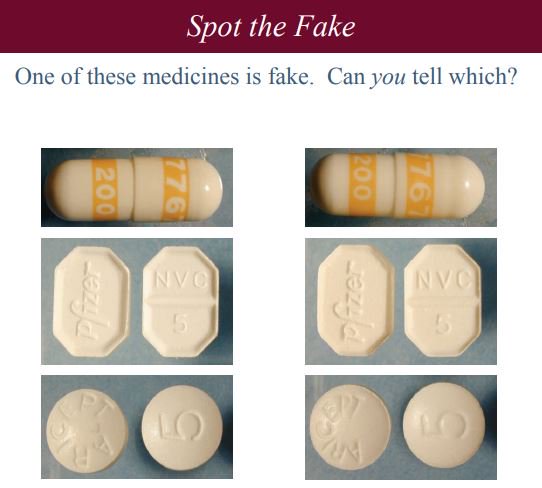The image features a maroon banner stretching across the top with the phrase "Spot the Fake" prominently displayed in white font. Beneath the banner, black text reads, "One of these medicines is fake. Can you tell which?" Below this text, the image is divided into two columns with a series of photographs on each side, arranged vertically.

In the left column:
1. The top photograph shows a white capsule with two yellow stripes. The top stripe is labeled "$7.76" while the bottom stripe says "$200."
2. The middle photograph displays a shape that resembles a cross between a hexagon and an octagon. On the left side of this shape is the word "Pfizer," and on the right side is the text "NBC5."
3. The bottom photograph depicts part of a pill. The visible part of the pill displays the text "A-R-C-E-P-T" on one side and the number "5" on the other.

In the right column:
1. The top photograph mirrors the image in the left column, showing an identical white capsule with yellow stripes labeled "$7.76" and "$200."
2. The middle photograph also resembles the shape in the left column with "Pfizer" on the left and "NBC5" on the right.
3. The bottom photograph is identical to the one in the left column, showing part of a pill with "A-R-C-E-P-T" on one side and "5" on the other.

Both columns of photographs appear nearly identical, making it challenging to discern between the real and fake medicines.